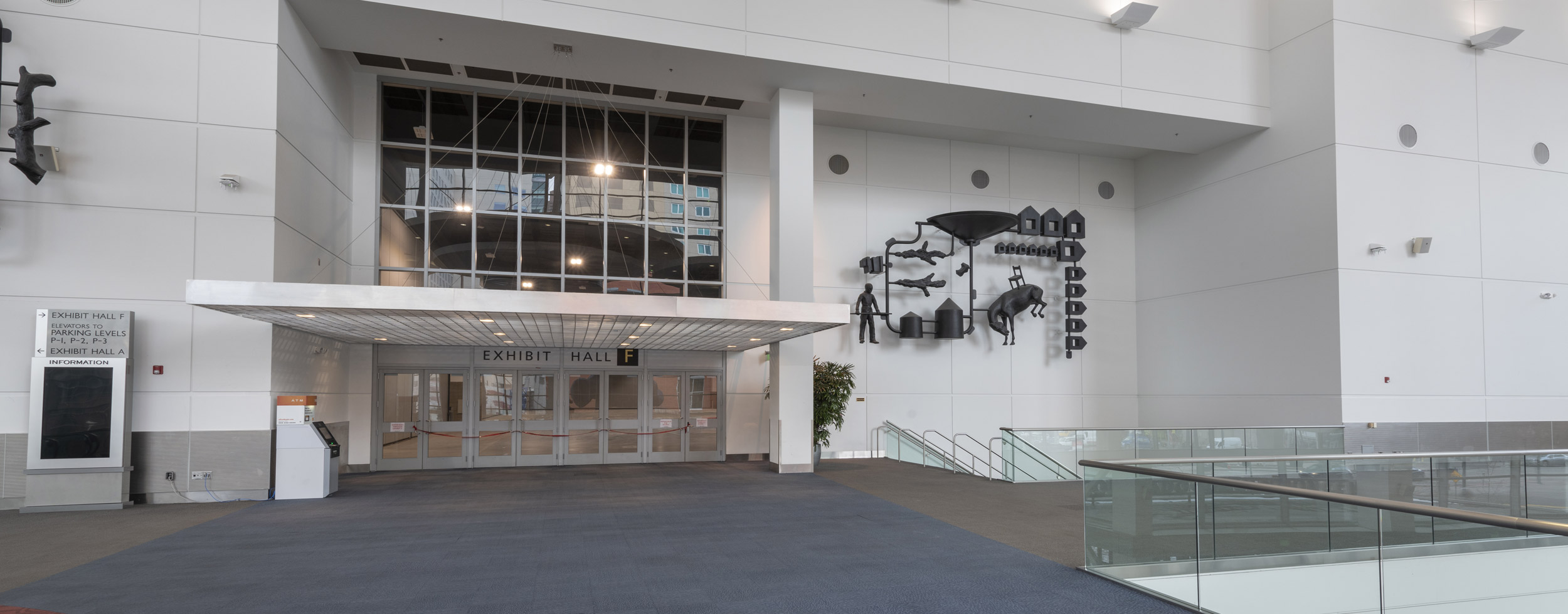The photograph captures the modern, white concrete exterior of a large civic building, which appears to be an exhibit hall or possibly a museum or convention center. The architecture features a blend of solid white paneling and extensive glass. The entrance is adorned with a large, horizontal porch roof, supported by strings extending to the top of the building. Below this canopy, a black (possibly blue) carpet leads up to three sets of doors, each marked with a red ribbon, and the inscription "Exhibit Hall F."

On the right side of the entrance, there is an intriguing sculptural wall installation, consisting of black metal structures that resemble a man, cylinders, an elephant, homes, and a funnel, adding an artistic flair to the otherwise modern setting. To the left, an electronic screen likely displays event information or ticketing services. Additionally, below the installation, a series of steps with glass railings lead downward, their destination not visible in the photograph. A large square column stands prominently near the entrance, contributing to the building's imposing and contemporary aesthetic.